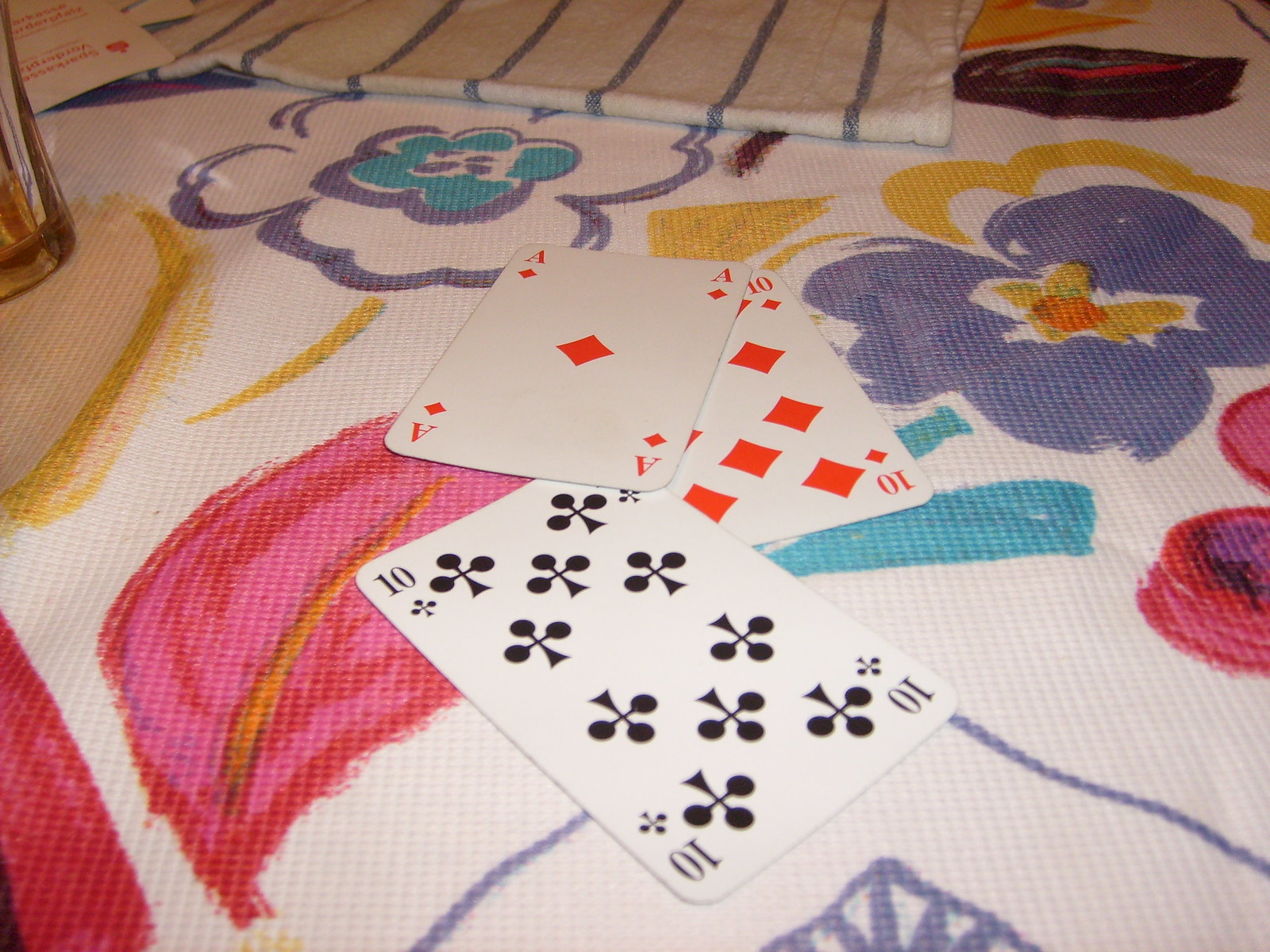On a delicately designed white tablecloth adorned with watercolor-style flowers, three playing cards lie spread out. The flowers are painted with intricate details: one flower exhibits a vibrant purple hue with a yellow center and yellow outlines, another showcases a blue center encircled by purple, leading to white petals outlined in purple, while a striking red leaf with a yellow spine features prominently in the lower left corner.

The playing cards displayed are the Ten of Clubs at the bottom, the Ten of Diamonds placed above it to the right, and the Ace of Hearts overlapping the Ten of Diamonds. The photograph is brightly lit, accentuating the vivid colors and fine details of both the tablecloth and the cards. Additionally, a white dishcloth with blue stripes drapes over the center top of the scene, adding a touch of casual elegance to the composition.